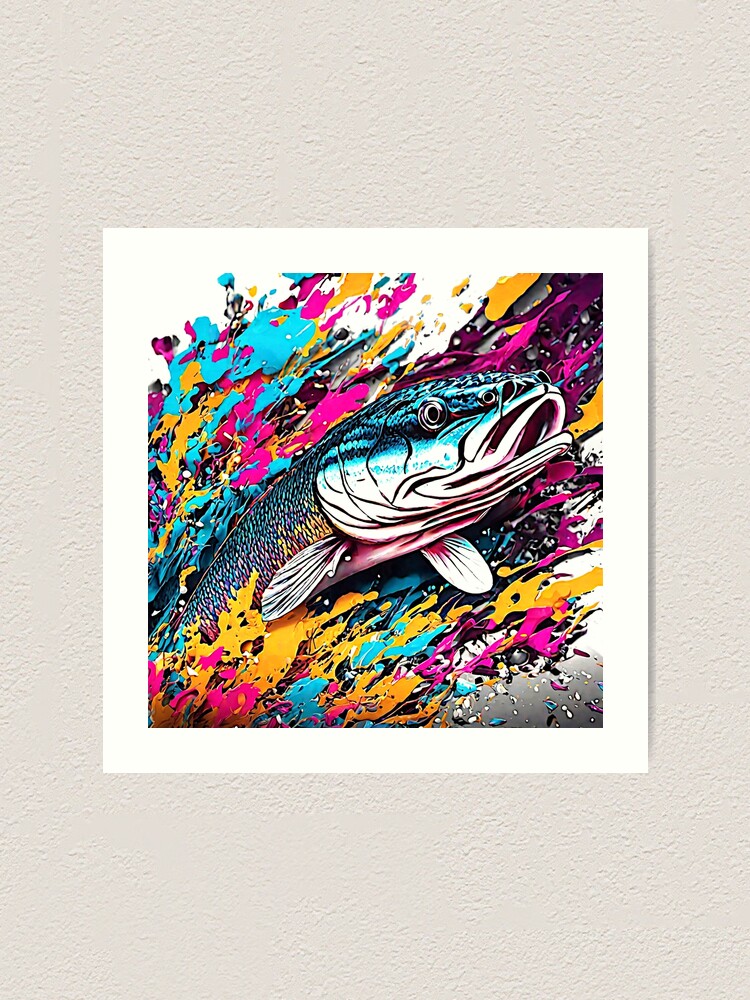In this rectangular cream-colored canvas, set against a textured white wall with visible marks, a vibrant stylized artwork captures attention. Dominated by splashes of bright blue, pink, and yellow paint, the piece features the dramatic side profile of a fish, possibly a carp or catfish, emerging dynamically from the colorful background. The fish, positioned centrally, faces right, displaying detailed scales that reflect the surrounding vivid hues. Its mouth gapes open, revealing prominent black eyes, whisker-like nostrils, and expressive gills marked by heavy black lines. The fish's front fins are visible, spread out beneath its head, while the tail remains out of view. The entire picture is encased in a white frame, enhancing the artwork's striking details and bold colors, which stand out against the beige backdrop.